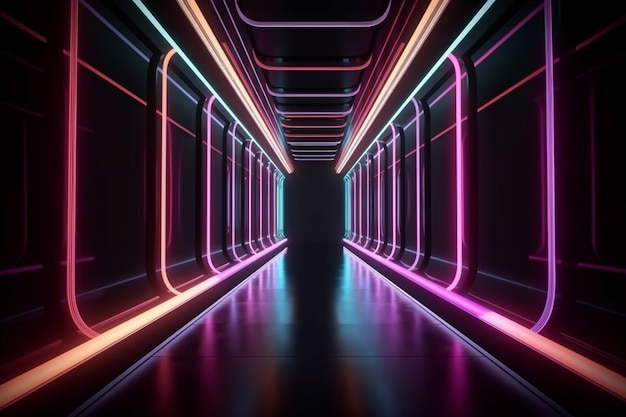The image features a strikingly modern hallway resembling the flamboyant aesthetics often seen in music videos. The floor, ceiling, and walls are all coated in a glossy black finish, providing a stark, dramatic backdrop. Lining the length of the hallway are several multicolored tube lights that add a vibrant, dynamic touch to the space. 

The floor of the hallway is accentuated with two long tube lights running parallel along each side. The tube light on the left side emits an orange hue that gradually blends into purple, while the right side features a pink light that transitions into purple. 

The walls also host an array of tube lights. On the left side, the lights are sequentially colored red, orange, pink, purple, and eventually blue at the end. In contrast, the right side showcases a progression of purple, pink, another section of purple, culminating in blue towards the end. 

The ceiling is adorned with a series of long tube lights arranged in various colors, with green, orange, and pink lights defining the space. Additionally, shorter crosswise tube lights intermixing purple and pink add to the visual complexity.

The overall effect is a dazzling corridor that feels both futuristic and cinematic, perfectly capturing the essence of vibrant visual storytelling.